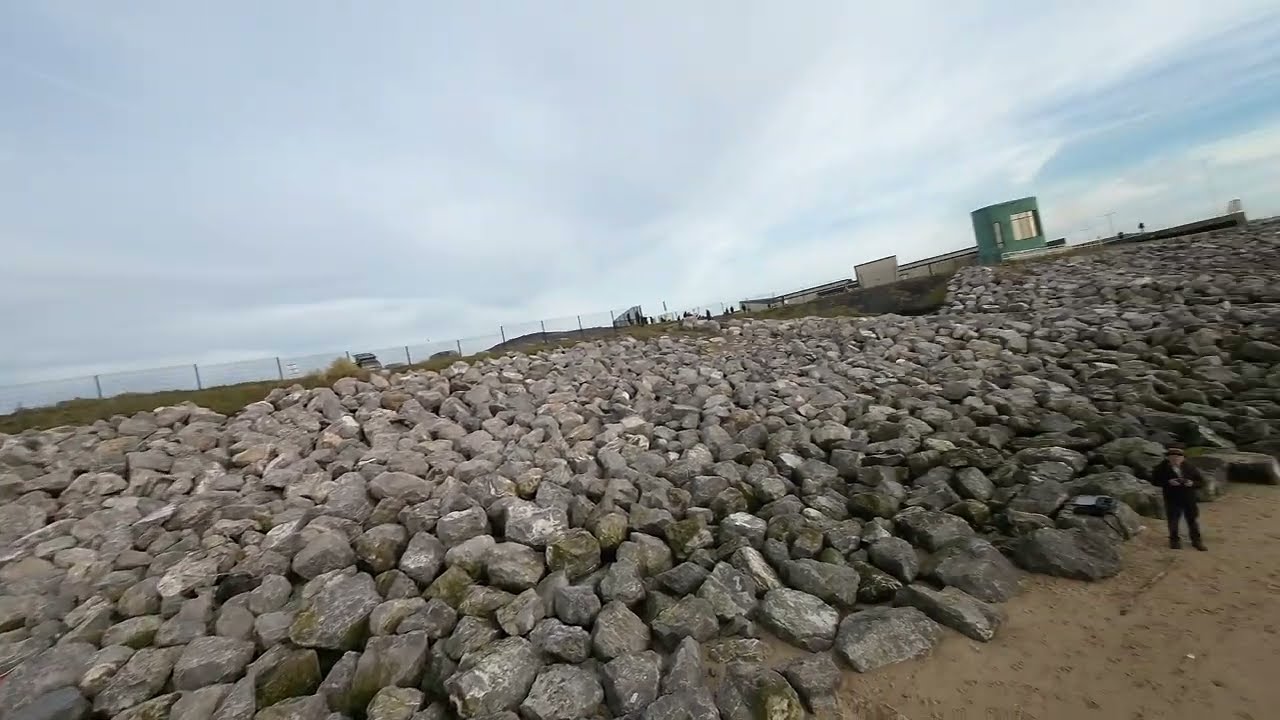In this landscape-style photograph, a man dressed in an all-black outfit, complete with a cap, stands on a patch of brown sand amidst a vast pile of large granite boulders, each approximately 6 feet in length and 3 feet high. These sizable rocks dominate the foreground, creating a rocky barricade that backs up to a hill topped with grass and bordered by a cyclone fence. The man has placed a bag on one of the boulders, and the overall scene suggests a barrier from the ocean, possibly a rocky beach. In the background, to the right, there's a green cylindrical structure in front of a flat-topped tan building, likely an industrial warehouse. The overcast sky is filled with white and gray clouds, with a small patch of blue in the top right corner. The photograph is slightly tilted, adding a dynamic perspective to the captured cloudy day.